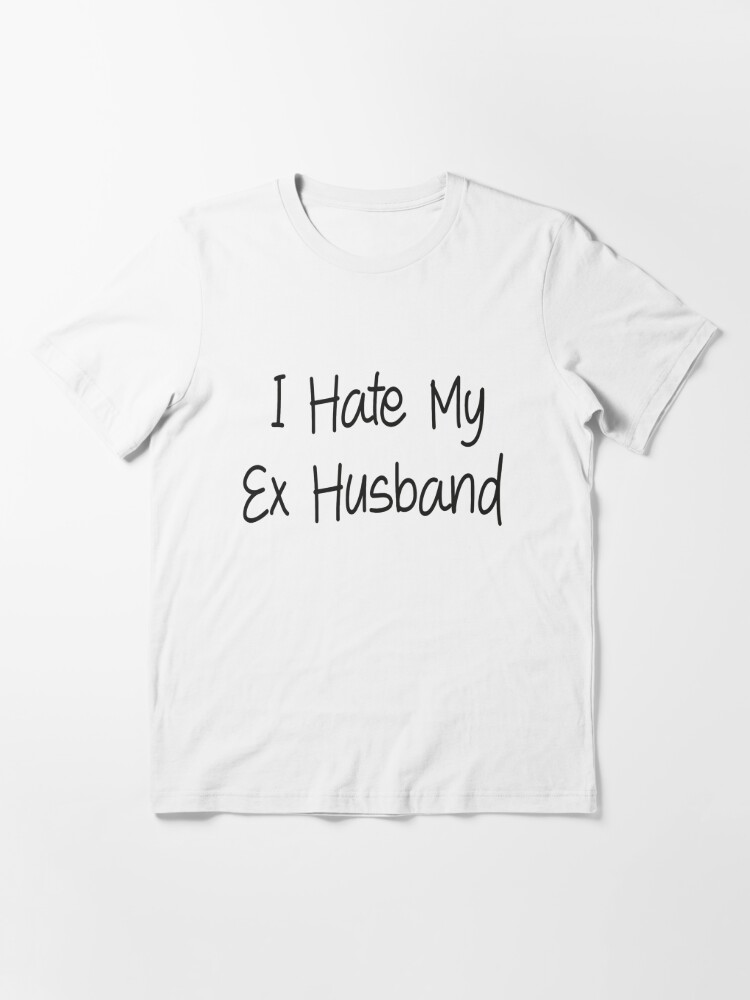This product image features a medium-sized, plain white t-shirt with short sleeves, meticulously laid flat on a white surface. The t-shirt bears the bold statement "I HATE MY EX-HUSBAND" in a distinctive, playful black handwriting-like font, with each letter fully capitalized. The t-shirt's sleeves appear slightly wrinkled but are otherwise laid out flat. Notably, the collar is free of any tags, emphasizing its simple, unadorned design. The well-made garment is centered in the image, casting faint shadows around its edges, and is devoid of any other colors or logos.